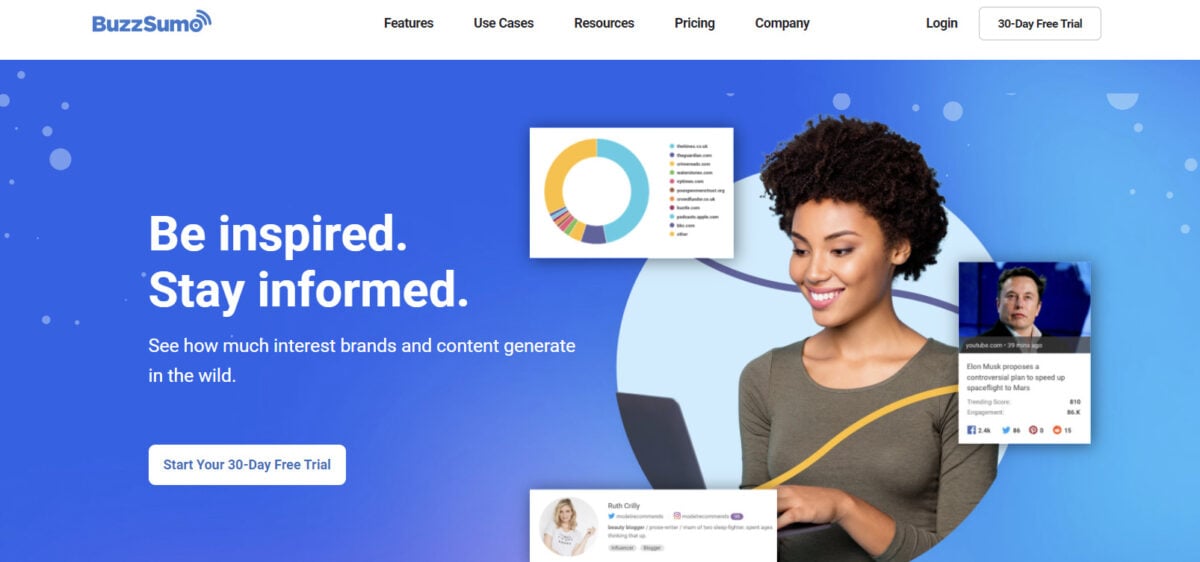This is a webpage screenshot featuring a striking central blue rectangular box with a blue background. The prominent white text within the box reads "Be inspired, stay informed." Beneath this, in smaller white font, the text explains, "See how much interest brands and content generate in the wild." Positioned below this text is a white button displaying blue letters that invite users to "Start your 30 day free trial."

To the right of the text, there is an image of a young, light-brown-skinned Black woman with natural afro hair. She is wearing a three-quarter sleeve olive green shirt and is radiantly smiling. The woman adds a warm, approachable element to the design with her chiseled chin and overall beautiful appearance.

Encircling her image, there are three graphical elements: a square on the right, two rectangles, and a circle. The square on the right side of the screenshot displays a picture of Elon Musk with an article snippet below it. To the left of her head is a circle that appears to represent some kind of budget plan. At the bottom, there is another element featuring an image of a white person (likely a woman) with text too small to decipher.

The top of the webpage features a blue header with the site name "BuzzSome" and menu categories labeled "Features," "Use Cases," "Resources," "Pricing," "Company," "Log in," and another button for the "30 day trial."